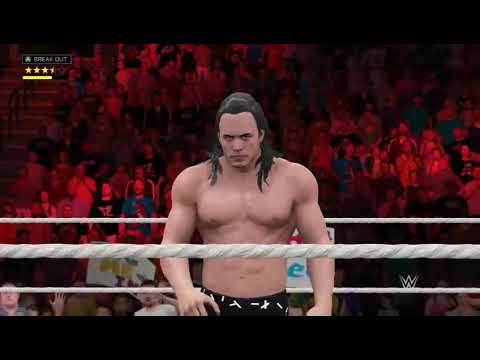A bold 3D graphic features the word "RAW" in striking red, block letters with a distinctive design where the end of the "R" extends beneath the "A" and "W." Each letter is outlined with a silver lining. This imposing text is flanked by spotlights above and below, casting their beams forward against a dark, black backdrop. The spotlights below rest atop a strip of black, while above them is a scaffold constructed of silver and gray pipes, giving the scene an industrial feel. The dramatic background showcases a fiery explosion in shades of glowing orange, yellow, and black, enhancing the intensity of the sign. On the left side, there appears to be a part of a WWE logo, underscoring the impression that this graphic is associated with a live wrestling event. The overall image has a captivating stadium-like ambiance, illuminated by the explosive display behind the centerpiece text.